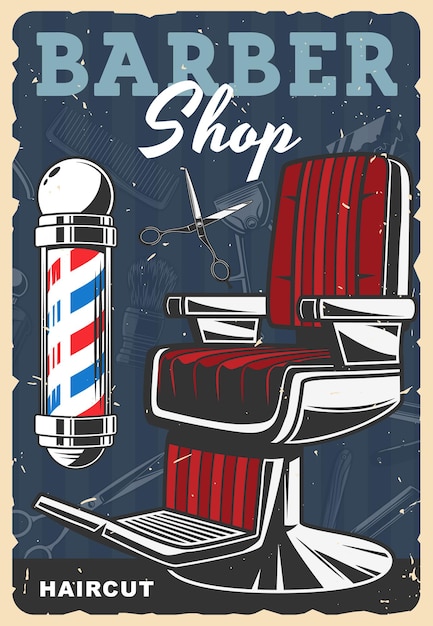This vintage barbershop poster features a meticulously hand-drawn design on a navy blue rectangular background with a subtle tan border. Dominated by a nostalgic aesthetic, the top of the poster prominently displays the word "BARBER" in large, light blue capital letters. Beneath it, "shop" is elegantly scripted in white, italicized font. Positioned on the left is an old-fashioned barber pole, complete with classic red, white, and blue diagonal stripes encased in a silver cylinder, topped with a round silver ball and a half-ball at the base.

Central to the image is a stately, vintage barber chair. The chair boasts deep red, almost burgundy cushioning on the seat and back, complemented by silver armrests, a silver footrest, and a wide, round silver base. Scattered across the navy blue background are ghosted images of grooming tools, including scissors, combs, and brushes, adding intricate detailing to the design. Between the barber pole and the chair hovers a floating pair of open, silver scissors, enhancing the thematic coherence of the scene.

At the bottom left corner, in all capital letters, "HAIRCUT" is boldly inscribed in white on a black bar, solidifying the poster’s call to action. The entire composition exudes a timeless charm, reminiscent of a bygone era, capturing the essence of traditional barbershops.